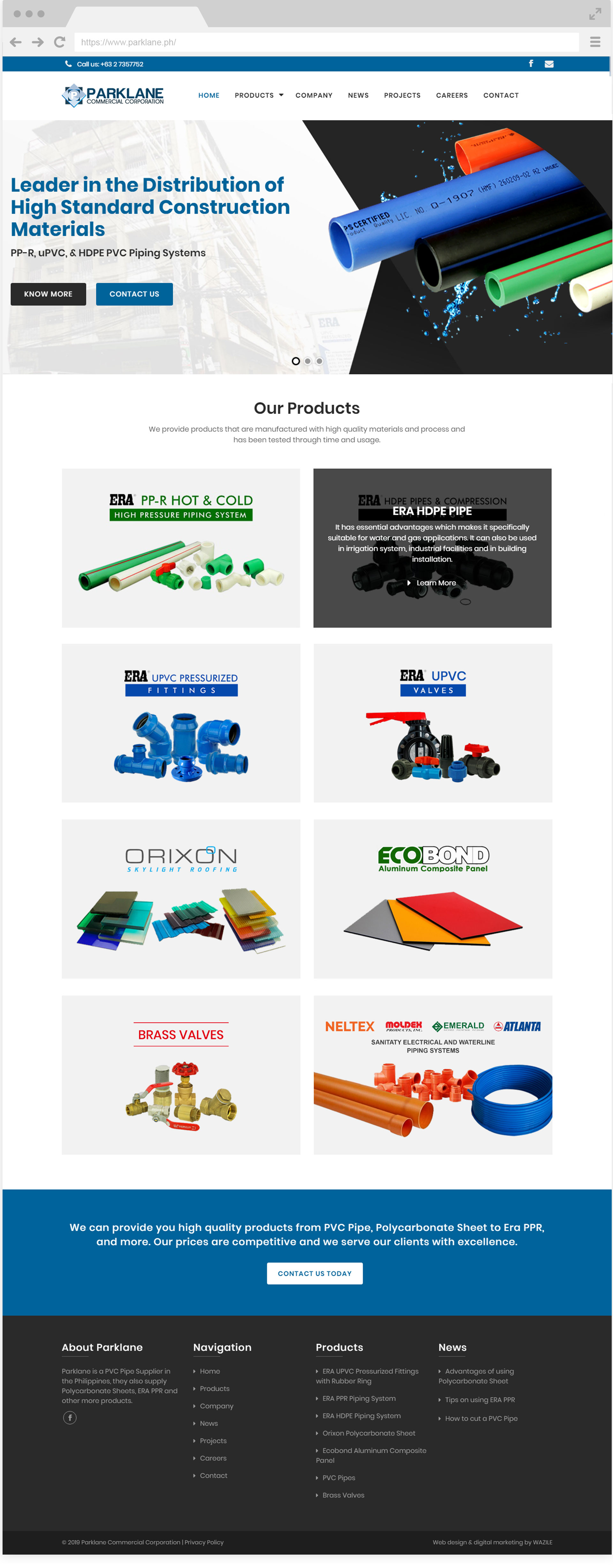This highly detailed image showcases a visually striking display of construction materials. Diagonally oriented across the frame, the composition features vibrant colors, including orange, blue, black, green, and white. These colors are represented as straws, implying variety in the types of materials presented.

The image is divided into six distinct squares, with an additional blue rectangle containing pertinent information about the products displayed and the website address.

- **First Square:** Displays a green and white straw amidst a scattering of green and white fragments, with a singular orange piece standing out.
- **Second Square:** Captures a collection of black and white straws and smaller pieces, emphasizing the diversity of materials.
- **Third Square:** Features three prominent blue tubes, showcasing the company's range of tubular products.
- **Fourth Square:** Contains a black cylindrical tube, highlighting another aspect of their inventory.
- **Fifth Square:** Depicts multiple slabs, suggesting a focus on flat, possibly modular materials.

Glitter and sparkling elements seamlessly merge throughout the image, adding an element of sophistication and drawing attention to the high standards of the construction materials on display.